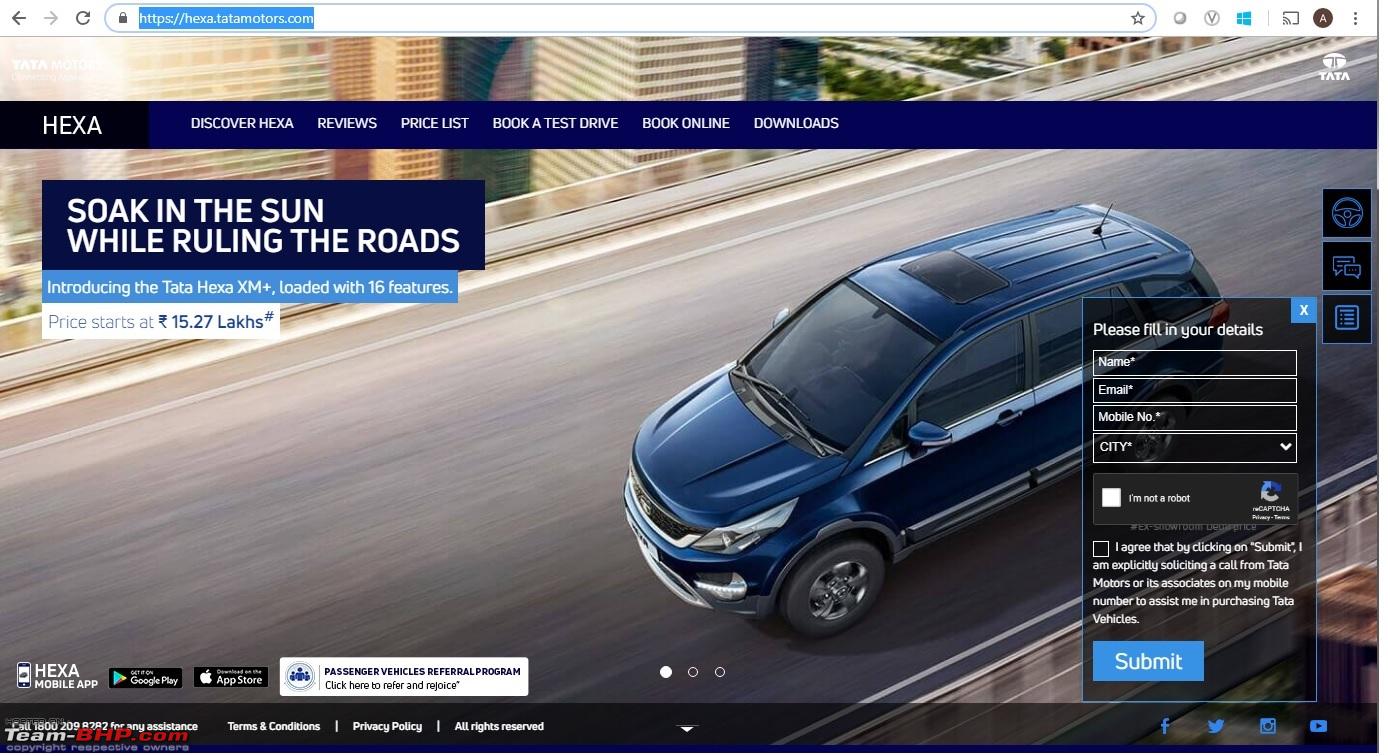The website represents a company called Hexa, as indicated by the black box with white text in the upper left corner that reads "Hexa." Adjacent to this box is a royal blue, horizontally-aligned rectangular bar that spans the entire width of the site. This bar features various hyperlinked categories in white text. The navigation options listed are: "Discover Hexa," "Reviews," "Pricelist," "Book a Test Drive," and another option starting with "Book," which is partially blurred and difficult to read, followed by additional blurred text.

Central to the homepage is an image of a vehicle resembling a minivan, suggesting that Hexa specializes in automotive products or services. Towards the bottom of the page, there are additional hyperlinks for legal and informational sections such as the Privacy Policy and Terms and Conditions. On the right-hand side of the screen, there is an information box where visitors can input their details to request more information about Hexa. This layout indicates a comprehensive and user-friendly interface for potential customers to explore the company's offerings and services.